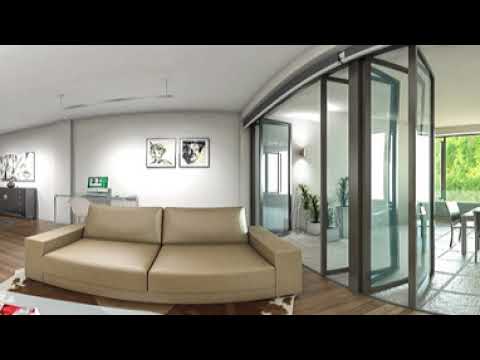The image showcases the interior of an apartment captured with a fisheye lens, giving it a distinctive rounded, bubbly effect. In the foreground, there are two light beige loveseats on a hardwood floor, facing a semi-transparent white coffee table adorned with a few magazines. A large animal skin rug sprawls beneath the seating area, with a smaller circular rug adding contrast. Mounted on the left side of the ceiling is an elegant wicker-style light fixture. The background reveals various apartment essentials, such as shelves of different sizes and photos along the wall. On the right, glass sliding doors lead to what appears to be a kitchen or dining area, identifiable by the table and chairs within. This adjacent room features tiled flooring and has two large windows, one of which is open, providing a view of lush greenery and trees outside.